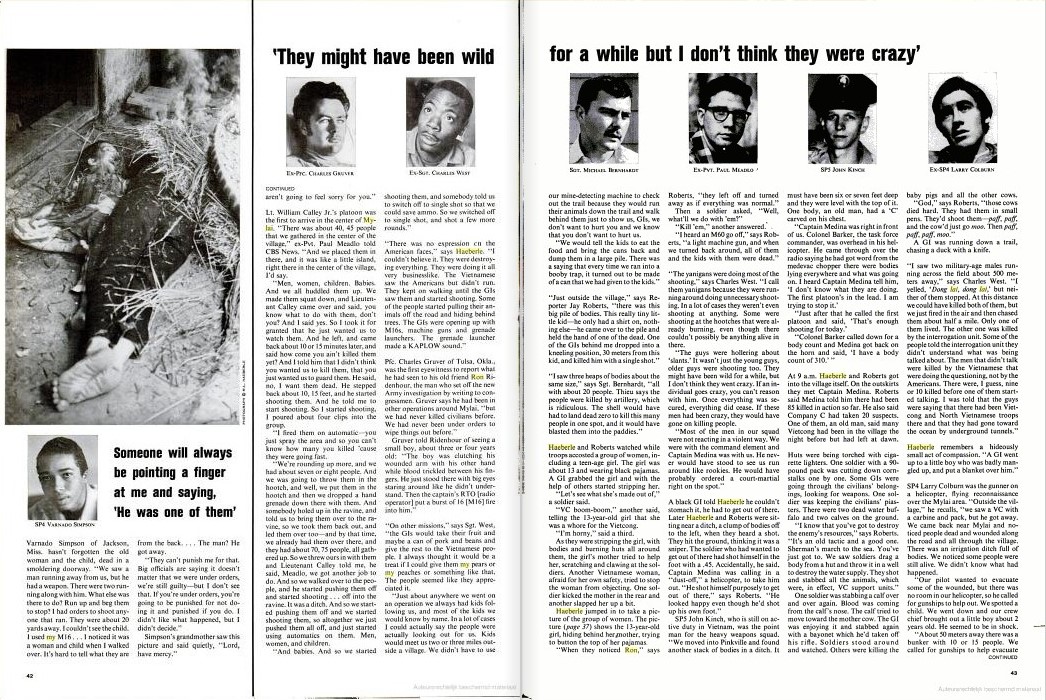This black-and-white image displays two adjacent magazine pages featuring a large, detailed article. The layout includes eight columns of text that are generally too small to read clearly. On the top of the left page, a shocking photograph shows the bodies of a child and an adult lying in front of a doorway, with hay scattered over them. Below this image, there is a quote in bold: "Someone would always be pointing a finger at me and saying he was one of them." Adjacent to this quote is a smaller picture of a young man. Above the text and to the right side of the page, there is another bold quote: "They might have been wild for a while, but I don't think they were crazy." Surrounding this quote are portraits of six men, spread across the top of both pages, identified by their names. The base of the pages is dominated by the extensive text of the article.